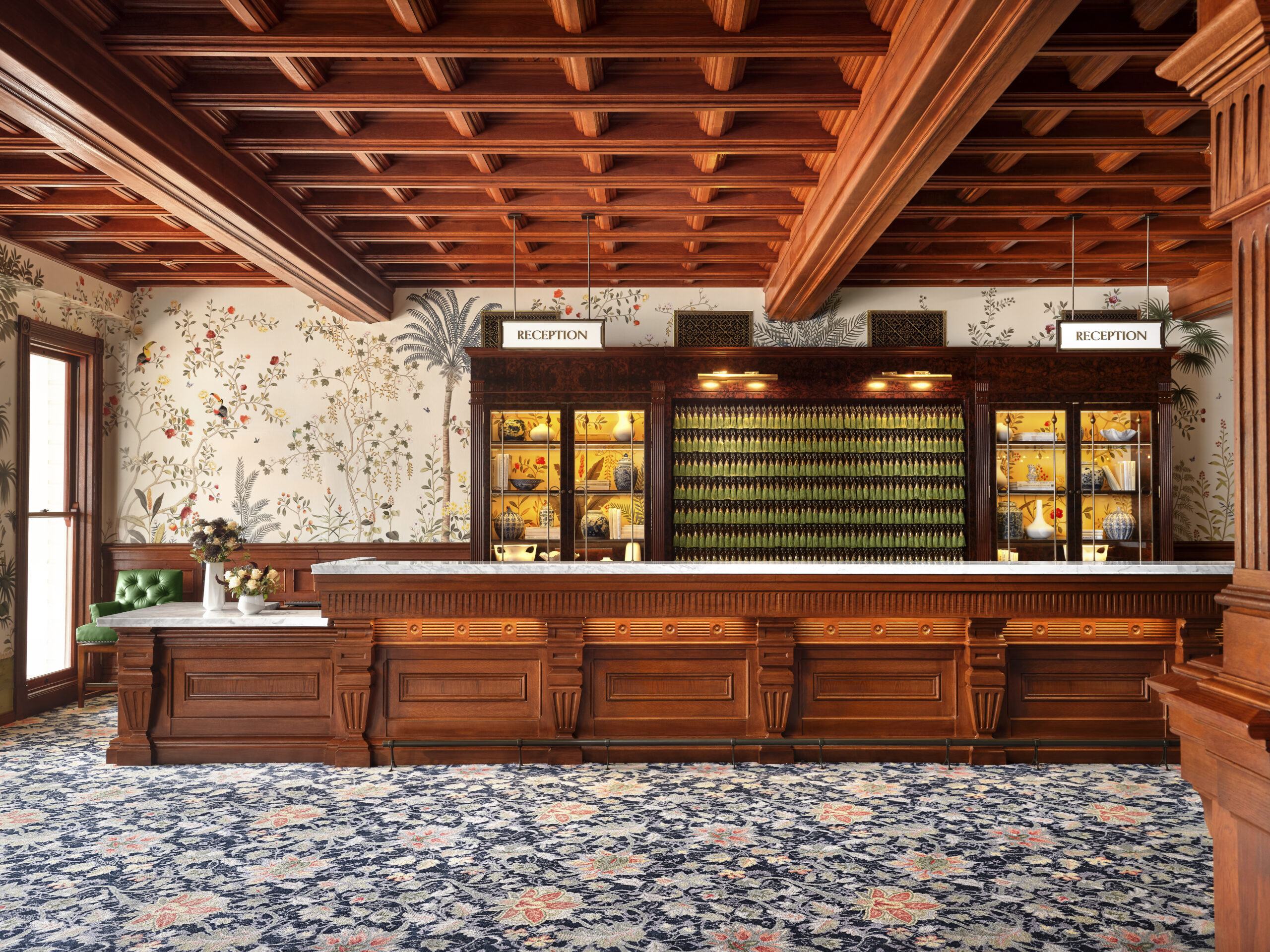The photograph depicts an elegantly designed old-school hotel lobby or reception area, showcasing meticulous attention to detail. The ceiling features an intricate wooden framework with horizontal, vertical lines, and elegant curves. The floor is adorned with a navy blue floral-patterned carpet, with white foliage and vibrant orange and yellow flowers. The central focus is a long reception desk, characterized by a dark wood base with intricate carvings and a contrasting white marble countertop. 

Two white rectangular signs reading "Reception" in black letters hang from the wooden ceiling. Behind the desk, there’s an ornate wooden cabinet displaying potteries and artifacts, illuminated by soft yellow lighting. The middle section of the cabinet houses rows of hanging green keys. A wooden case flanking the cabinet holds glass shelves, also lit up with a warm yellow light. To the left, a door emits a bright white light, adding a modern touch to the otherwise classic ambiance.